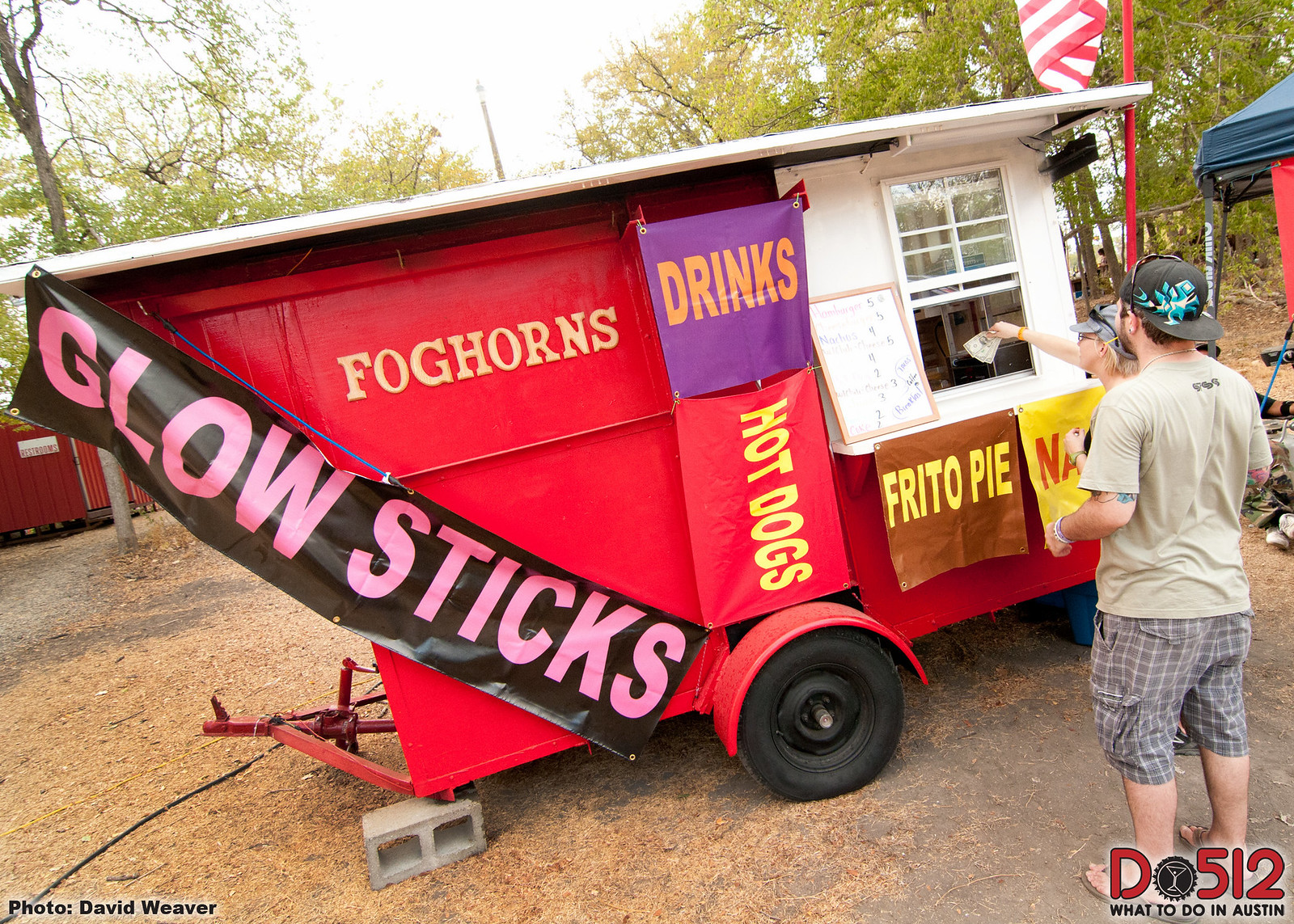In this image, a red pickup truck converted into a food truck is parked in an outdoor, wooded area. The truck is adorned with several signs advertising items such as glow sticks on a black background with pink text, fog horns, hot dogs, Frito pie, and drinks. People are gathered at a window, placing their orders. The surroundings include dirt and scattered wood chips on the ground, and a mixture of concrete flooring is also visible. A man wearing a T-shirt, shorts, and a backwards hat stands in the bottom right corner. Trees populate the background, and a flag is visible against the sky, indicating an outdoor setting in the middle of the day. The scene is filled with various colors including red, black, pink, gray, light brown, yellow, orange, and green, centering around the bustling food truck.